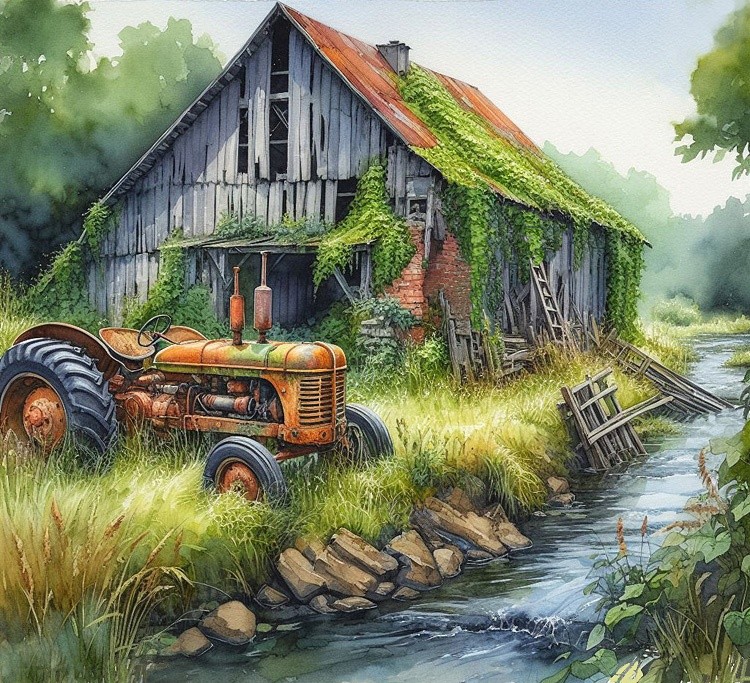The artwork is a detailed, animated painting of a dilapidated, abandoned barn or farmhouse set in a desolate countryside. The once-functional structure is now falling apart, with openings and gaps visible throughout its old, whitewashed wooden planks. The barn features a V-style metal sheet roof overrun by green vines and weeds, matching the overgrown grass and vegetation surrounding it. In front of the barn, there's a vintage tractor from the 1930s or 1940s, originally painted green but now mostly rusted with large tires in the back and smaller ones in the front. A fast-flowing stream with dark blue-green water runs beside the building, bordered by scattered rocks and wooden debris from the barn. The sky above is hazy, adding to the sense of abandonment, and there's a hint of a tree in the upper right corner. This evocative scene, which seems to have been painted either digitally or with traditional mediums like acrylic or oil, captures the serene yet melancholic beauty of nature reclaiming a forgotten piece of history.